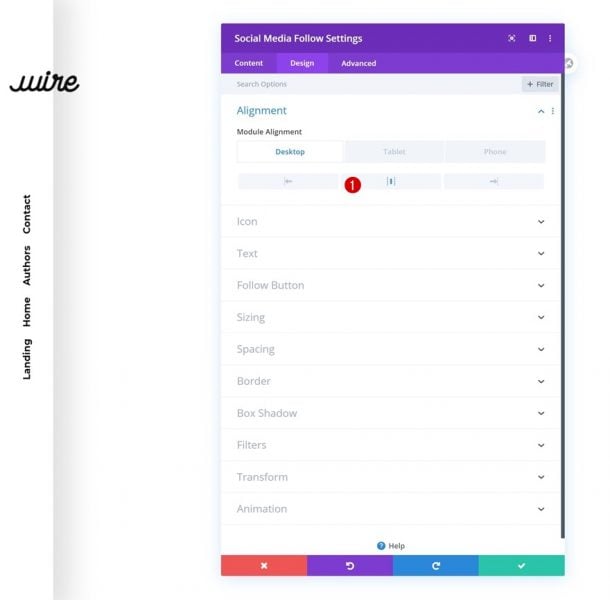The image depicts a website interface identified as "WIRE," indicated by a cursive black text logo positioned in the top left corner. Along the left-hand side, there is a vertically oriented menu containing options labeled "Landing," "Home," "Authors," and "Contact," requiring viewers to tilt their heads slightly to read.

Dominating the center of the screen is a heading bar with a purple background that reads "Social Media Following Settings." Within this bar, there are several functional tabs named "Content," "Design," and "Advanced," accompanied by a search bar and a filter button situated just below.

Beneath the heading bar, the subtitle "Alignment" with the subtext "Module Alignment" is present, offering interface options for various devices: Desktop, Tablet, and Phone. The Desktop option is currently selected. Additionally, there are numerous drop-down menus available for customization, including but not limited to Icon, Text, Follow Button, Sizing, Spacing, Border, Box Shadow, Filters, Transform, and Animation.

At the bottom of the screen, there are utility buttons for Help, Undo, Redo, and Save, as well as an X button for closing the window. The interface is designed to offer extensive customization and navigation features for users managing their social media settings.